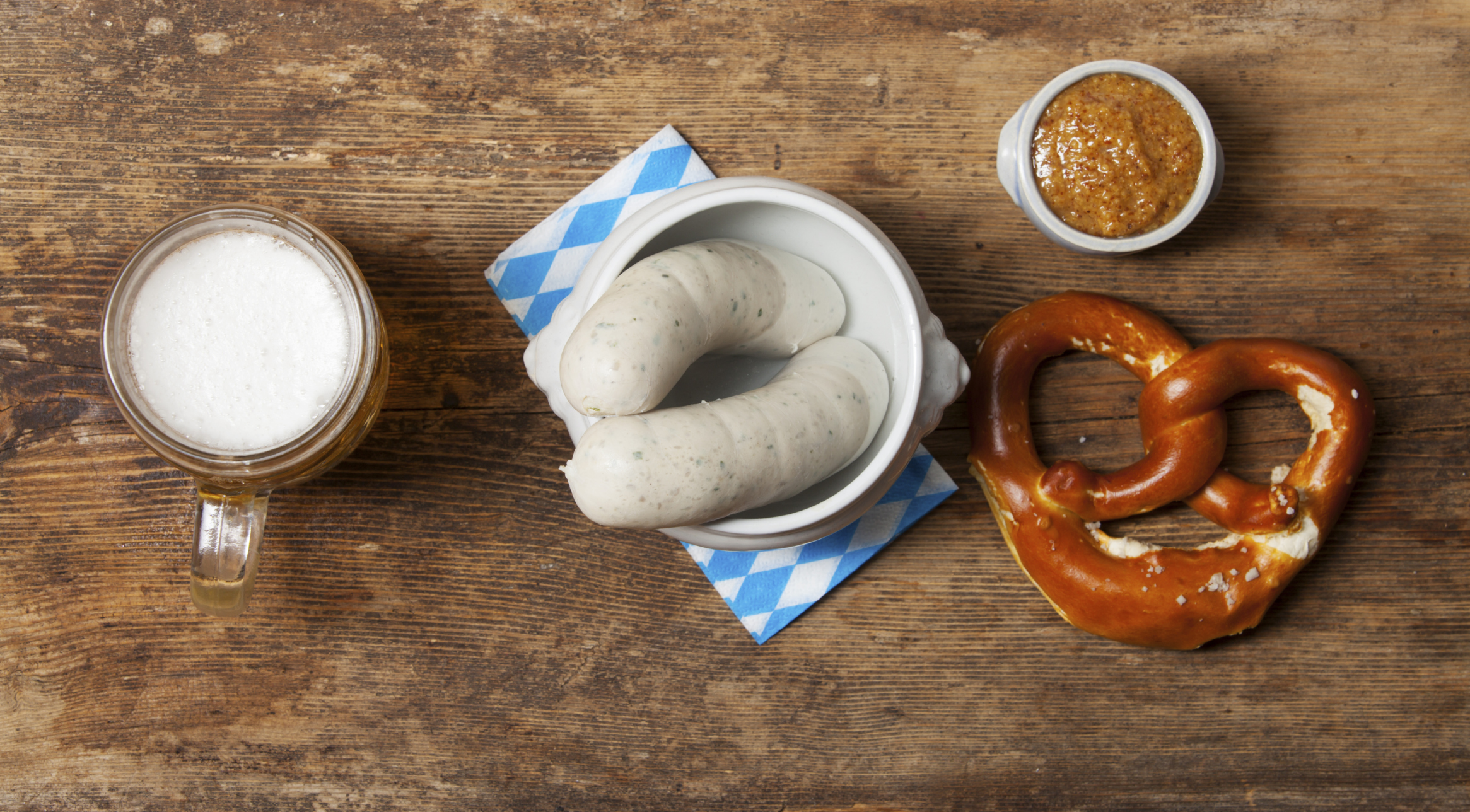This high-quality image presents an appetizing food layout on a rustic wooden tabletop captured from a top-down perspective. Dominating the center is a white bowl with handles, cradling two white sausages speckled with black flecks, perhaps suggesting they are uncooked or delicately prepared. The bowl rests on a white napkin adorned with blue diamond patterns. To the left, there's a clear glass mug filled with golden beer, topped with a frothy white head. On the right side of the sausages, a freshly baked pretzel with a glossy brown exterior, likely just out of the oven, sits invitingly. Positioned above the pretzel is a white ramekin containing what appears to be a mustard-style dipping sauce, completing the enticing arrangement designed to appeal visually and gastronomically.